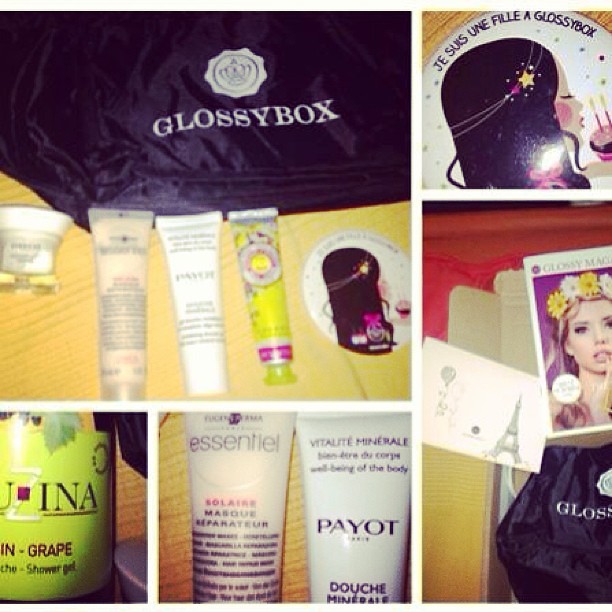The image is a photo montage composed of five distinct tiles, each providing a glimpse into various beauty products and promotional items, all tied together by the theme of "Glossy Box." The largest tile prominently features a purple velvet bag with "Glossy Box" inscribed in white letters. Below the bag are a small cream canister and three beauty product tubes labeled as INA Grape, Essential, and Payoff. On the top right, there's a card with an illustration of a woman with black hair blowing out birthday candles, accompanied by the text “Je suis une fille, a Glossy Box.” Towards the bottom, close-up shots highlight the mentioned products in more detail, though slightly blurred. In the bottom right tile, there's an actual photograph of a woman adorned with a flower crown. The entire montage is interspersed with French text, adding a sophisticated and international touch to the presentation.